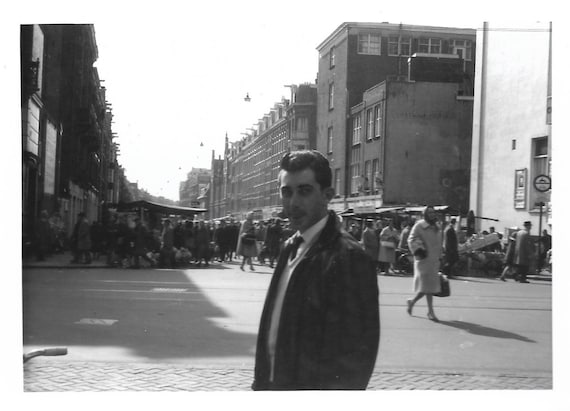This detailed black-and-white photograph, likely from the 1950s, captures a bustling city street scene. At the center, a man with a pompadour hairdo, dressed in a button-down shirt, tie, sweater, and jacket, gazes mysteriously at the camera. He is slightly turned to the left. Surrounding him are busy streets with three to four-story buildings lining both sides. To the far left, a sidewalk hosts multiple people walking past a building. On the far right, a woman in a long coat holding a suitcase can be seen casting a shadow ahead of her. The background reveals more people, giving a sense of a crowded haymarket or bus stop area, and one can spot several flags or banners fluttering from the tops of buildings. Additionally, some distant objects hovering in the sky could be interpreted as helicopters or lights, adding an intriguing element to the photograph's urban landscape.